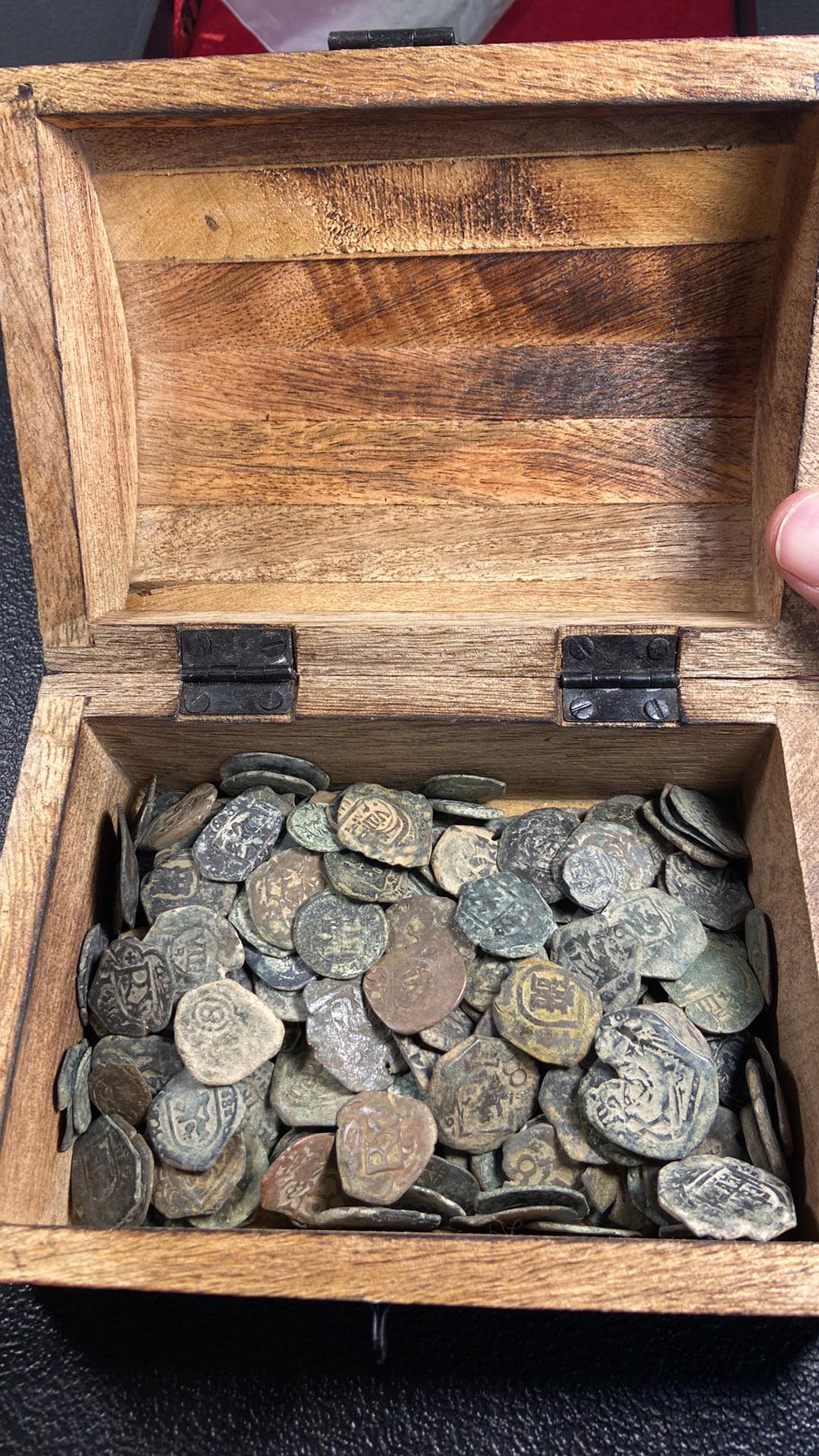The image depicts an open, handmade wooden box brimming with a multitude of old, hand-pressed coins. The box, featuring two dark gray or black hinges secured with flat-head screws, is held open by a person’s thumb visible at the left edge of the frame. The coins, numbering approximately 200, display a variety of colors ranging from brown and gray to light green, indicative of a patina formed over time. Many of these coins are round, while others are slightly misshapen, and all appear worn and caked with dirt, obscuring the intricate carvings on their surfaces. The lid's construction reveals individual wood pieces glued together, and a latch mechanism is visible at the front. This chest, nearly filled to the brim, rests on a black tabletop with hints of red and white peeking through at the background's upper edge.